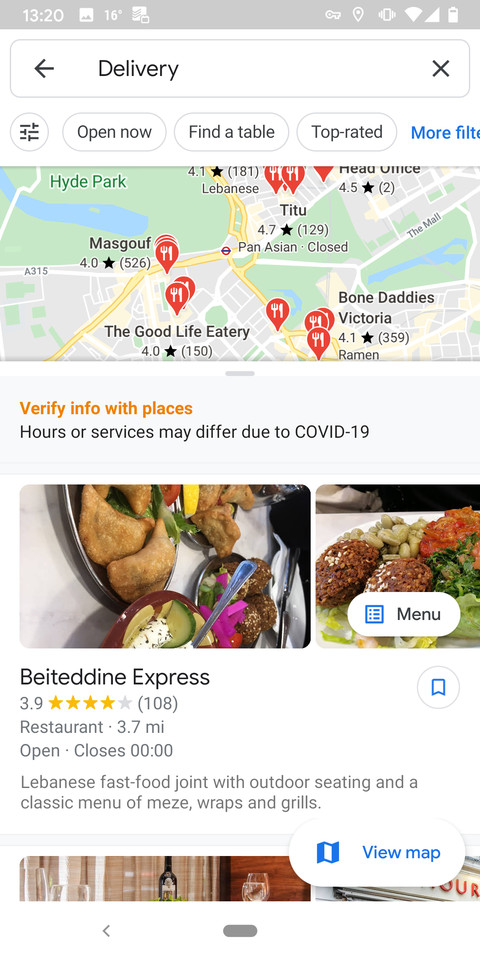A detailed screenshot from a mobile device, likely a phone, showing the screen dimensions. In the status notification bar at the top, it displays the time as 13:20. The temperature is 16 degrees, the battery is at 80%, and both cell signal and Wi-Fi are fully strong. The device is in silent mode, and location services are active.

The open application appears to be Google Maps, featuring a clean white background. The user has searched for "delivery" in the search bar at the top. The map layout is filled with numerous red pins, each bearing a knife and fork icon, indicating different restaurants that offer delivery services in the user's vicinity.

The foremost restaurant listing is "Betadine Express," boasting a rating of 3.9 stars out of 108 reviews. It is located 3.7 miles away. The description highlights Betadine Express as a Lebanese fast food joint featuring outdoor seating and a traditional menu, including various mezze, wraps, and grills.